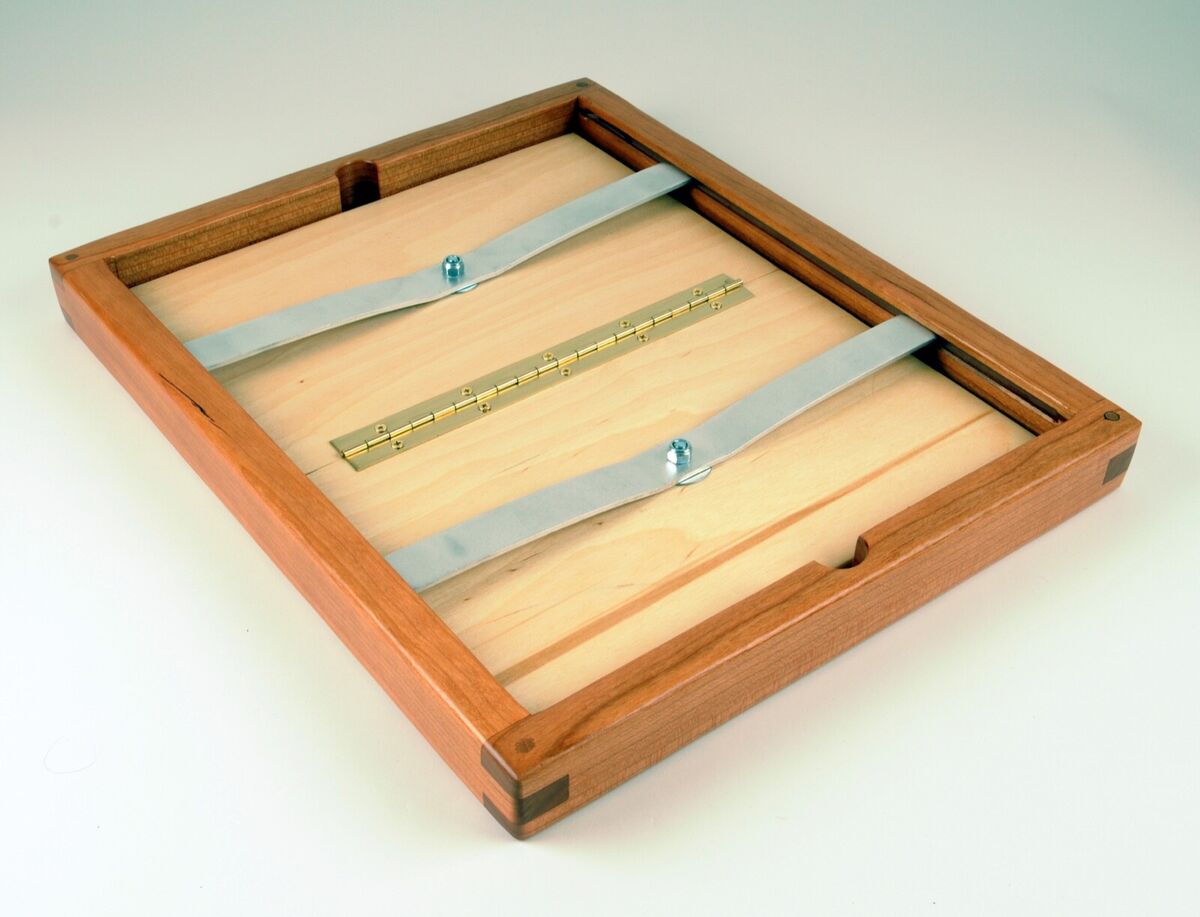The image depicts a wooden rectangular box, positioned diagonally over a versatile, ombre background that transitions between different shades of gray, adding depth to the scene. The box itself features a blend of rich cherry wood on the exterior and lighter wood on the inside. It is engineered with a hinge across the middle, indicating it can fold in half. The hinge is gold and complemented by silver steel strips that flank each side of the hinge, secured by bolts, enhancing the box's structural integrity. This careful detailing suggests it is not merely ornamental but functional.

The box is set on a plain white surface which contrasts nicely with its wooden texture. Each corner of the box showcases darker wood that reinforces the edges, adding a touch of character and durability. Notably, the box contains two marbles inside, both blue, and positioned within small carved-out grooves at the top and bottom. These marbles suggest a gameplay element, potentially involving flicking or maneuvering them towards a goal, reminiscent of classic board games.

Overall, the visual harmony of the cherry and light woods, combined with the practical design of gold and silver metallic components, highlights both the aesthetic and functional design of this intriguing board game box.